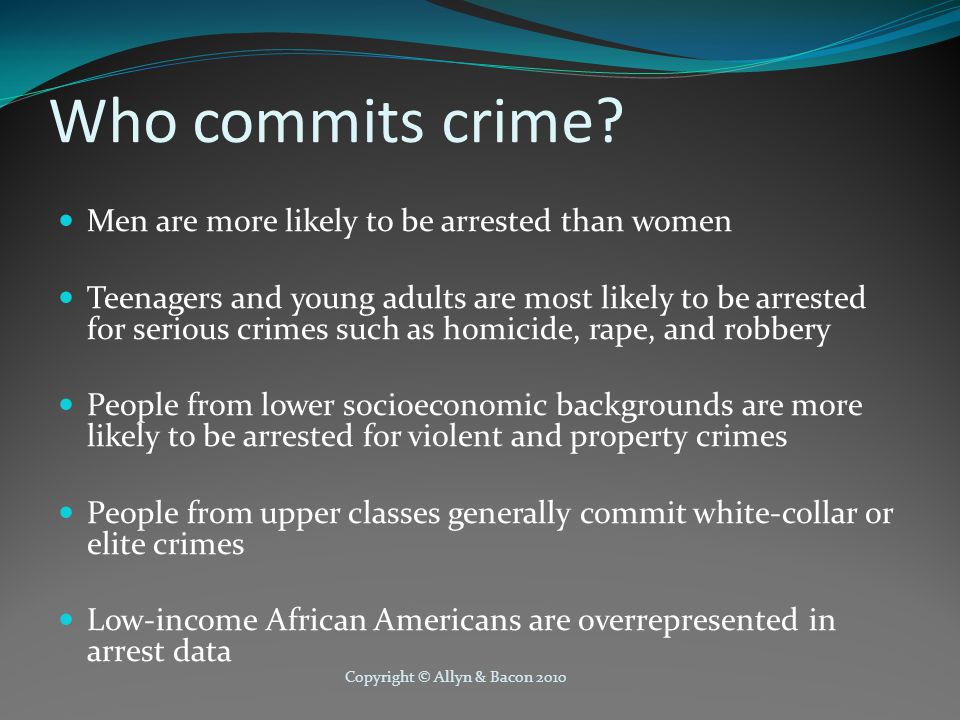The image features a significant amount of text against a predominantly solid blackish-gray background, with a decorative swirl of alternating blue and black lines at the very top. Centered at the top of the image is a white heading posing the question, "Who commits crime?" Below this, several blue bullet points with white text detail various crime statistics. The points are as follows: men are more likely to be arrested than women; teenagers and young adults are most likely to be arrested for serious crimes such as homicide, rape, and robbery; people from lower socioeconomic backgrounds are more likely to be arrested for violent and property crimes; people from upper classes generally commit white-collar or elite crimes; and low-income African Americans are overrepresented in arrest data. The image concludes with a small-font copyright notice at the bottom, stating "© Allen and Bacon 2010." There are no images or icons, just text against the solid background.